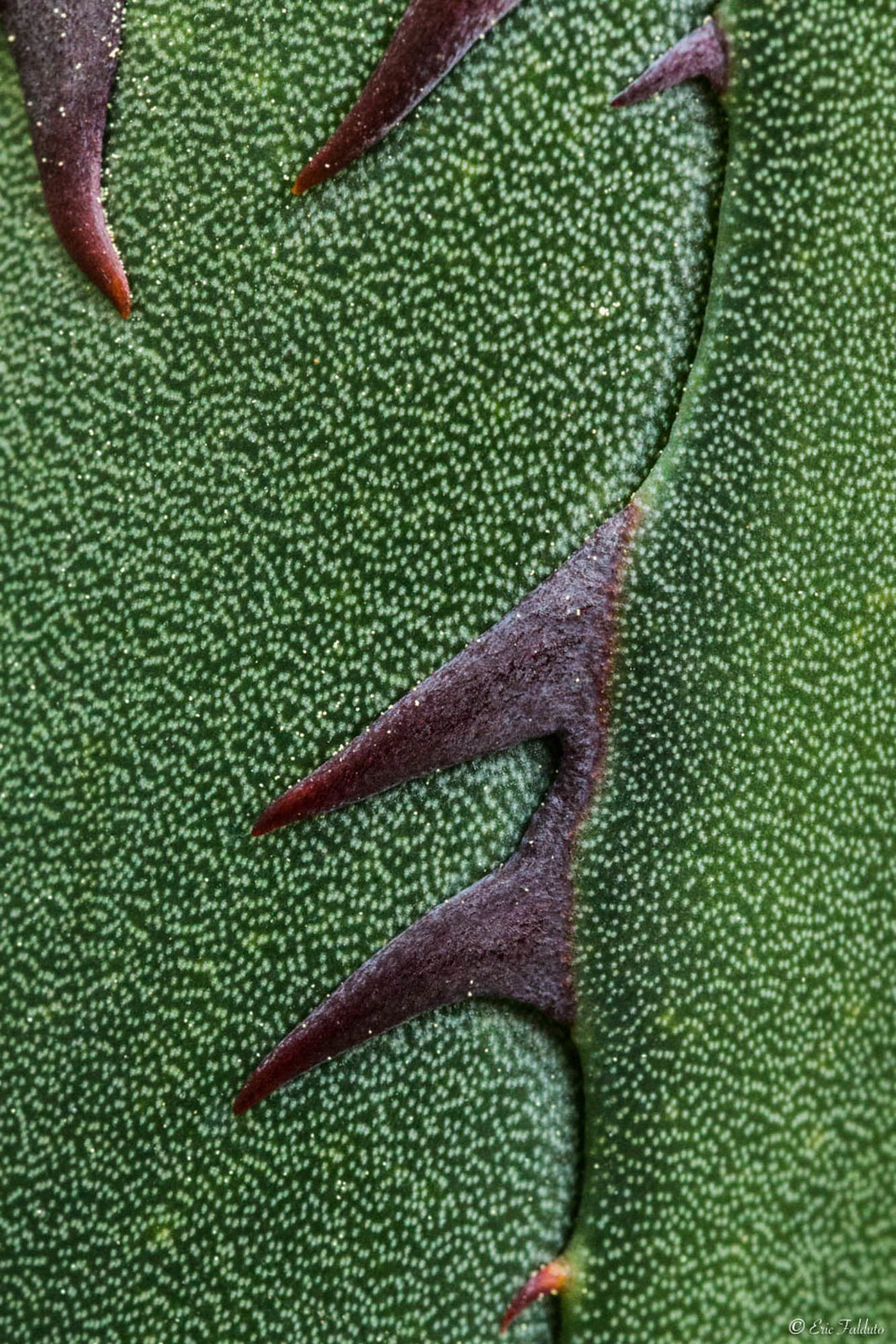This image, possibly an abstract painting or a highly detailed photograph, depicts a mysterious and captivating scene that merges naturalistic and surreal elements. The background is primarily dark green, punctuated by lighter green and almost white dots, creating a speckled, textured effect that suggests either a field of grass or an aquatic surface rippled with reflections. The central motif features a series of gray, sharp-edged structures resembling fins, potentially from a mythical sea creature or reminiscent of thorns on a plant. The largest and main fin-like element runs vertically with three distinctly positioned fins, where the top one is smaller, and two larger fins are in the middle. To the left, two more incomplete fins are visible, their tapered ends cut off at the image’s edge. Near the bottom, an orange tint highlights a smaller fin, adding a contrasting warm hue to the composition. The details incline towards a realistic interpretation, such as a close-up of a thorny plant, but their otherworldly sharpness and arrangement hint at a deliberate abstraction by the artist. Clarity comes from the lower right, where a signature and copyright text read possibly as “Eric Taylor” or a similar name, anchoring the piece in the realm of intentional artistry.